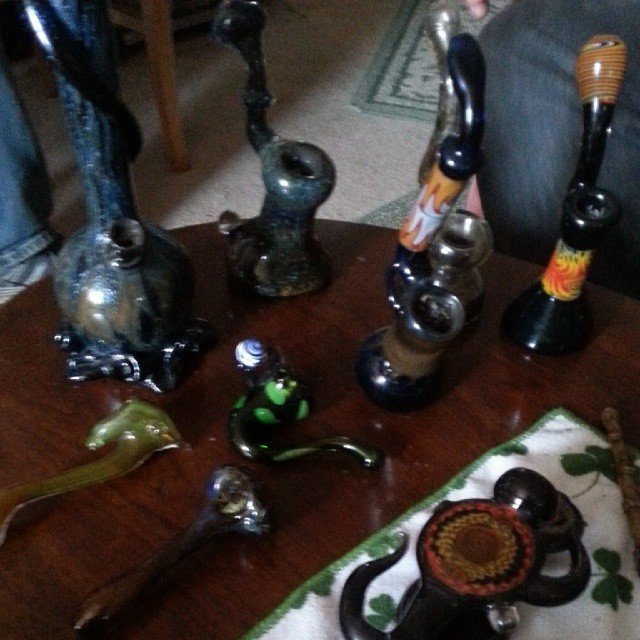In this image, we have a detailed scene featuring a collection of decorative smoking devices displayed on a dark brown, glossy wooden table, likely enhanced with an epoxy coating. The table has an almost square shape and sits in a living room setting. There are various smoking pipes and bongs, including a medium blue bong and several intricate glass pipes of different colors – including blue with brown bases, orange and white, yellow, green, and dark green. Some of these pieces appear fragile and ceramic-like, with unique shapes and ornaments.

On the table, to the bottom right, lies a white cloth adorned with green shamrocks, and one of the smoking utensils is placed on it. Additionally, there are several small bowls scattered around the lower half of the table.

In the background, a pinkish carpet is visible, topped by a green and cream-colored rug. The scene is further animated by two individuals partially visible; one is wearing blue jeans and shoes, positioned on the left, and another set of jeans is on the right. There's also evidence of a wooden chair and table legs, suggesting a cozy, lived-in space.

The combined elements of colorful, intricate bongs, and pipes along with the casual arrangement of furniture and cloths create a vivid tableau of a unique and personal collection.